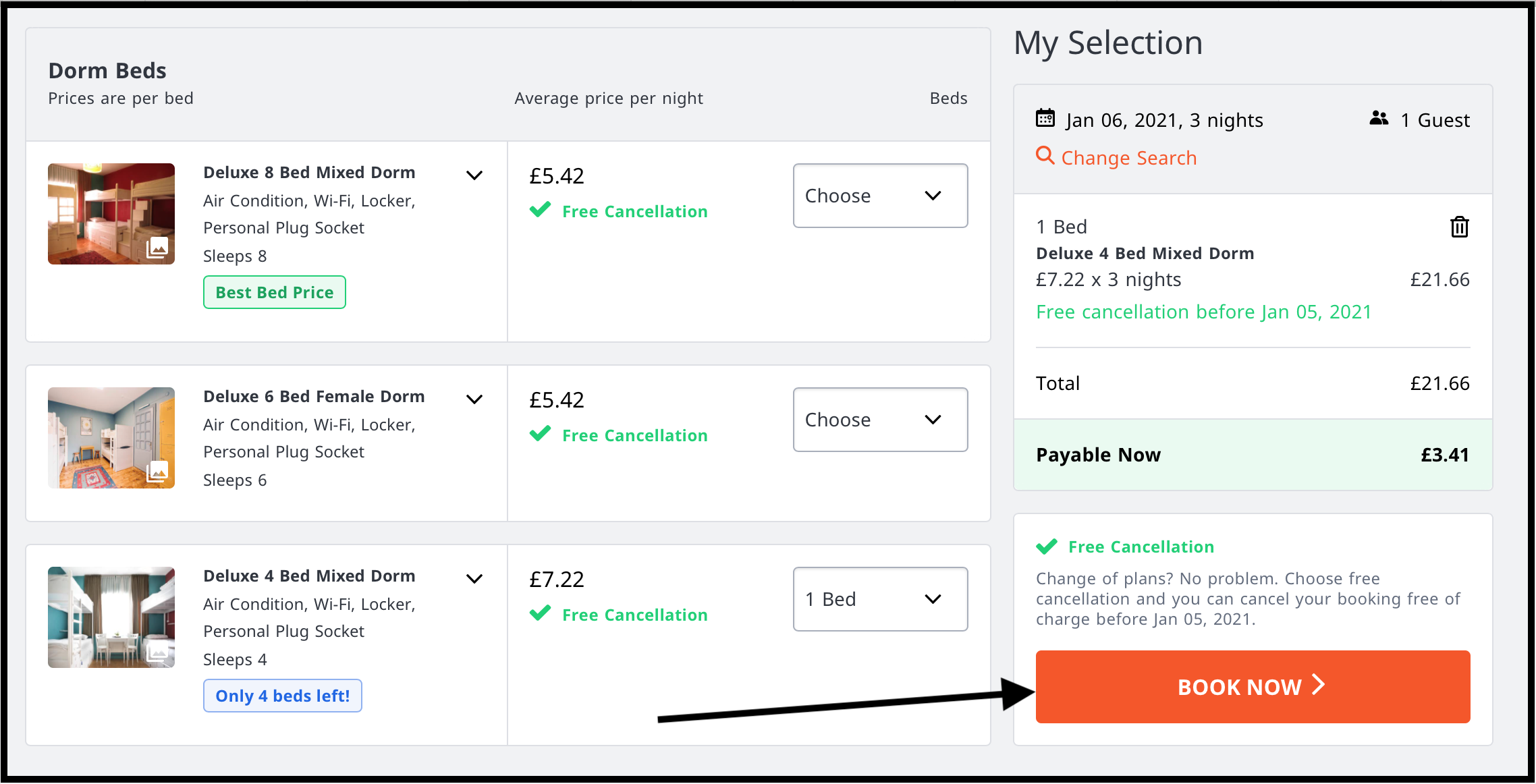The web page for booking accommodation is displayed on a horizontal rectangular screen with a light blue background and a black border. In the upper left-hand corner, the bold text "Dorm Beds" is prominently featured, with the smaller gray text "Prices are per bed" beneath it. To the right, there is text indicating "Average Price per Night" followed by "Beds."

Below, there are three horizontal white boxes, each containing an image of the respective room on the left and a detailed description. The pricing is listed in pounds (£), not USD. 

The first box describes a "Deluxe 8-Bed Mixed Dorm," and includes details such as "Air-conditioned," "Wi-Fi," "Locker," "Personal plug socket," and "Sleeps 8." Beneath this description, there is a green button labeled "Best Bed Price" in green text. To the right of this, the price is listed as £5.42, accompanied by a green check mark and the notation "Free Cancellation" in green text.

Similar detailed information and layout are provided for the remaining selections. In the bottom right-hand corner of the page, there is a large orange button with white text that says "Book Now."